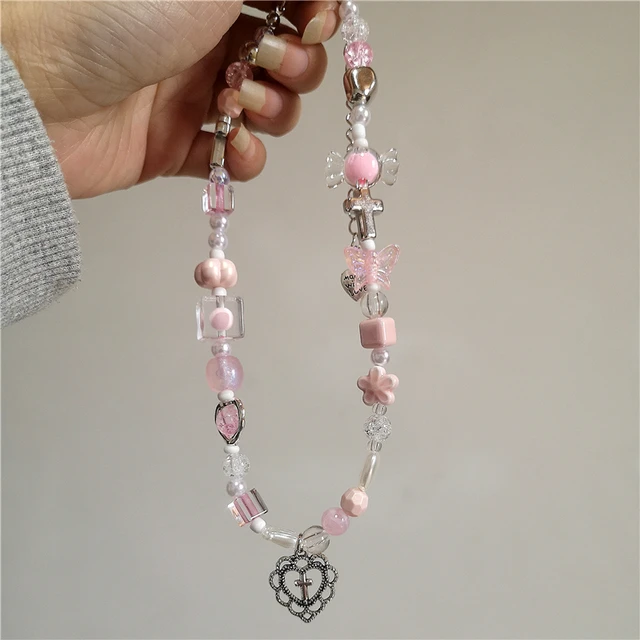This color photograph, shaped square with a pale gray or tan background and subtle shadowing, prominently features the left hand of a woman in the upper left corner. Her long, manicured nails and the gray cuff of her shirt or sweatshirt are visibly detailed. The woman's thumb is out of the frame, but her palm and folded fingers elegantly clutch a handmade rosary that cascades down to the bottom of the image. This rosary, adorned with a mélange of clear and pale pink glass beads, includes cube-shaped beads, round beads, and ornamental ones reminiscent of candy wrappers or angel wings. The rosary is further decorated with pink butterfly beads, smaller pearlescent spacer beads, and a few faceted peach-colored beads, alongside a distinct five-petaled flower-shaped bead. At its terminus, the rosary features a noteworthy pendant depicting a sacred heart with a cross at its center. The intricately designed necklace, measuring approximately eight to ten inches in diameter and strung with a mix of beaded shapes, blends both aesthetic appeal and spiritual symbolism.